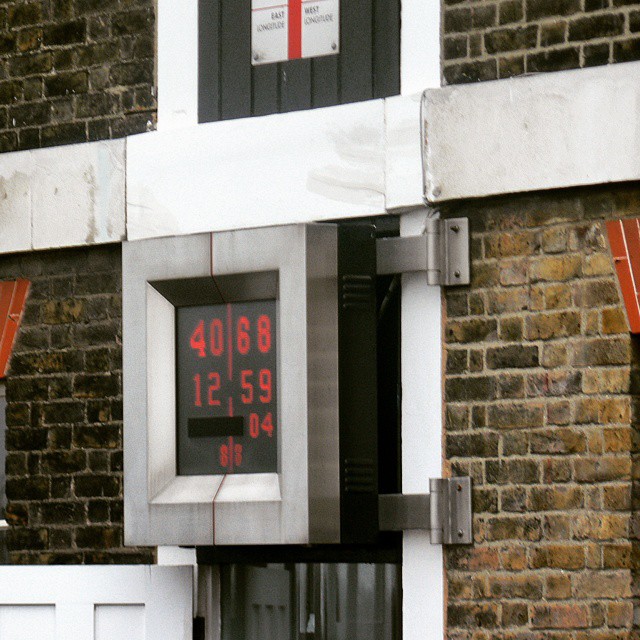This image showcases the exterior of a brick building, focusing on a prominent sign with various details. The sign is encased in a thick, gray outer border. Centrally displayed on the sign is the number sequence "4068125904," with the number "88" situated below it inside a black, sideways rectangle. This rectangle features a silver-colored, box-shaped border. To the right of the sign, there are two gray hinges attached to a white post. Above this white post is a horizontally aligned rectangle that includes gray and white sections. The building itself is constructed of brown bricks, and at the very top of the image, there is a black pattern overlaid with a red crossing design and small black text. Finally, in the bottom left corner of the image, part of a white door is visible.